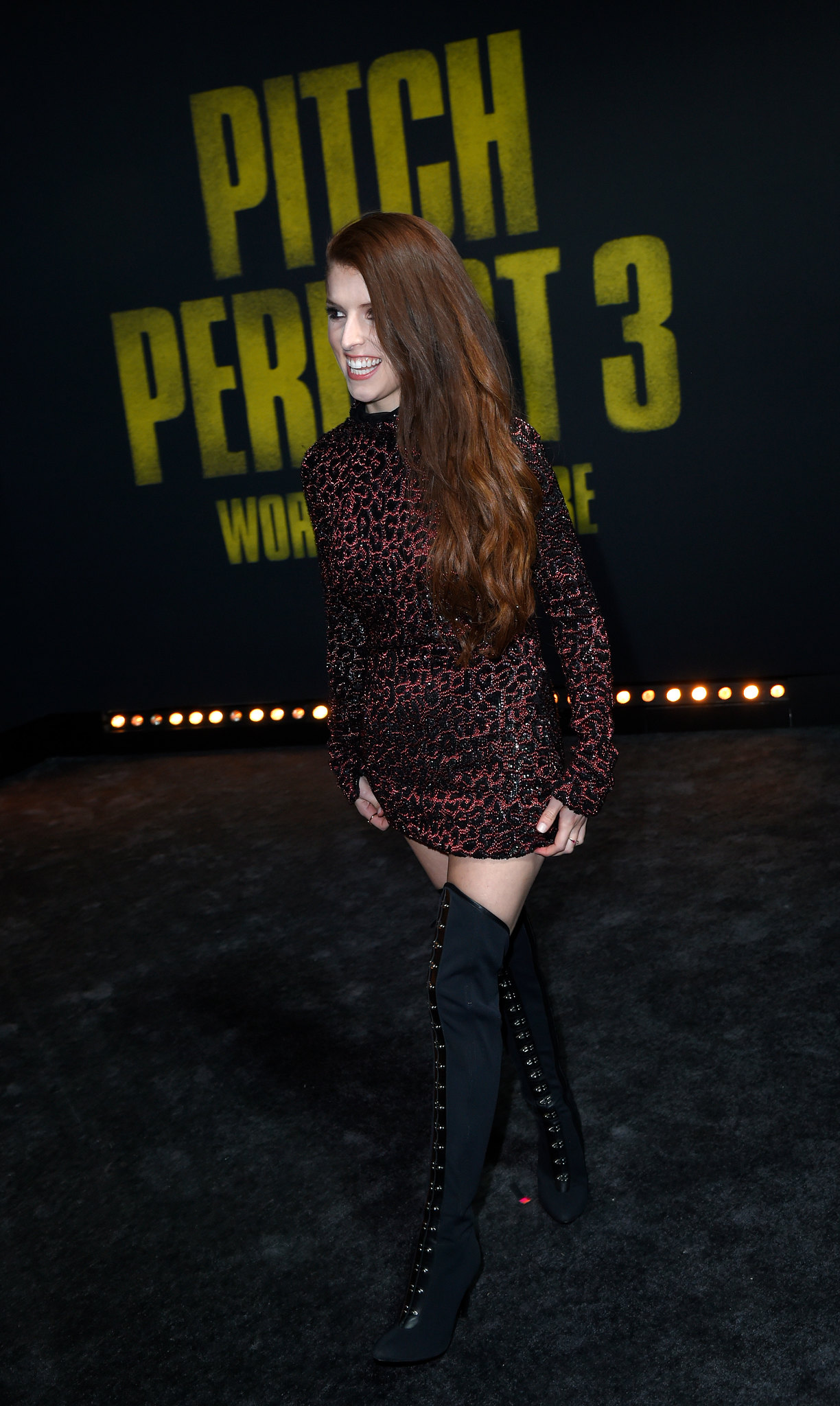In this full-color nighttime photograph taken at a movie premiere, an actress is striking a pose on a dark carpet, likely to be a black or very dark shade. The backdrop is dominated by a large, black banner emblazoned with bold, yellow letters that read "Pitch Perfect 3," illuminated by small lights at the bottom. The banner also features the text "World Premiere." The actress is centered in the frame, in sharp focus, and she exudes charisma with a wide, open-mouthed smile as she gazes towards the left corner of the image.

She is adorned in a long-sleeved, sequined dress featuring a black and red leopard print design that ends at her waist. Complementing her outfit, she wears striking knee-high black felt boots, adorned with gold jewelry that travels up to her thighs. Her long, reddish-brown hair cascades down to her midriff, and she enhances her appearance with lipstick, emphasizing her fair complexion. Her stance, with one foot slightly in front of the other, adds a dynamic feel to the image, capturing the glamour and excitement of the movie premiere event.